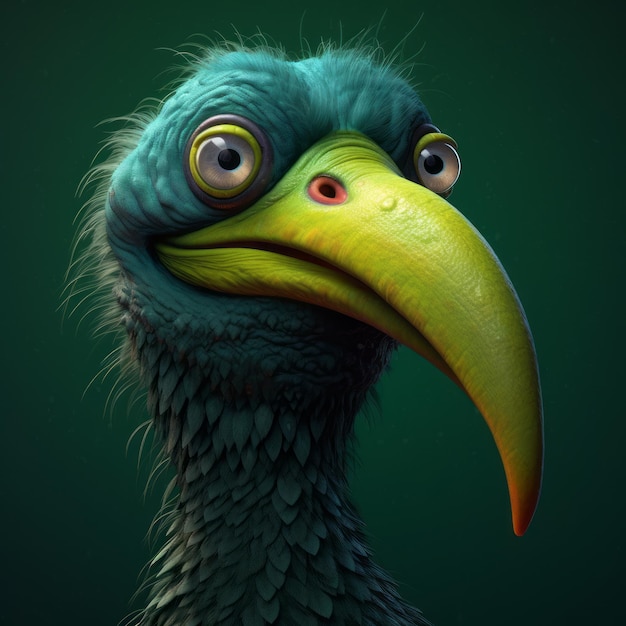The detailed image depicts a vibrant, cartoonish bird with a uniquely long, curved, and pointed beak that transitions from yellow-green to an orange tip, featuring an orange nostril hole. The bird’s eyes are strikingly bulging, reminiscent of googly eyes, encircled by a chartreuse green ring followed by a purple ring. Its head and neck are adorned with plentiful, feathery wisps that resemble thin, fluffy fibers, creating a textured appearance with a blue-green to teal hue. The backdrop of the illustration harmonizes with the bird’s color, maintaining a sea green to emerald green tone. This meticulously crafted, AI-generated or digitally drawn artwork focuses closely on the bird’s neck and head, highlighting the intricate, short feathers and delicate strands that catch the light, making the bird’s portrayal appear both detailed and lifelike.